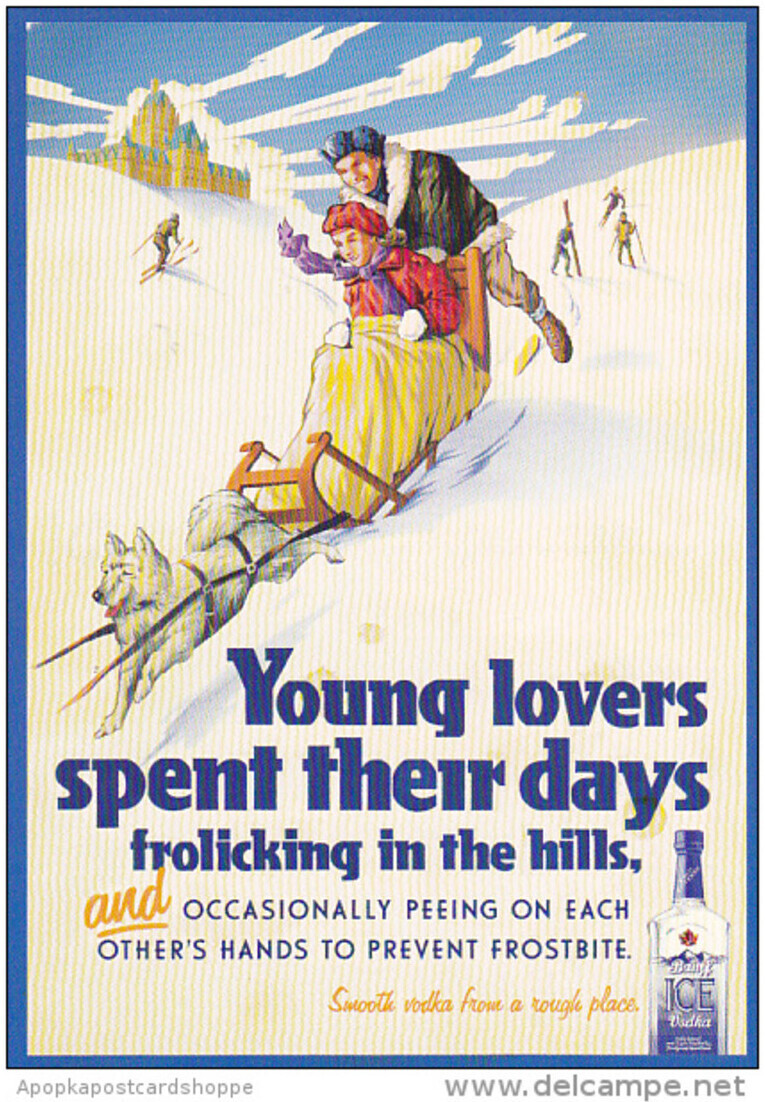The image appears to be a nostalgic advertisement for vodka, styled like an old-school postcard with a blue border. The central artwork, possibly computer-generated or cartoony, depicts a winter scene under a beautiful blue sky with scattered clouds. In the background to the left, a castle or large orange building with a blue roof sits atop a snowy hill. In the foreground, a romantic winter activity unfolds with a couple: a woman wrapped in a yellow blanket, wearing a red jacket, purple scarf, and gloves, sits on a sled. A white dog is pulling the sled forward, while a man in a green jacket, beige pants, and boots pushes from behind. Additional figures can be seen skiing in the background. The bottom of the image features bold blue text declaring, "Young lovers spend their days frolicking in the hills and occasionally peeing on each other's hands to prevent frostbite," accompanied by the tagline in yellow, "Smooth vodka from a rough place." A bottle of vodka is prominently displayed on the right-hand side. The bottom of the image also includes text like "Apop Cap Postcard Shop" and "dellcamp.net," suggesting it may also serve as a postcard. Yellow stripes decorate the scene, adding a whimsical touch to the festive and vintage atmosphere.